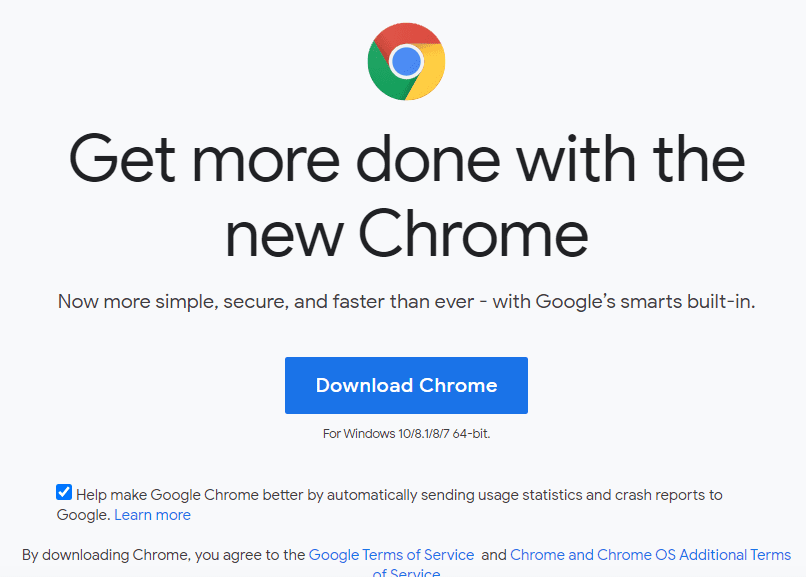The image depicts the download screen for the latest version of the Google Chrome Browser. At the center-top of the screen, the iconic Chrome logo is prominently displayed, featuring its distinctive red, yellow, and green outer segments encircling a blue circle at the center. Directly below the logo, in large black font against a grey background, is the headline: "Get more done with the new Chrome." 

Beneath this, in a smaller font, there’s a message stating: "Now more simple, secure, and faster than ever, with Google's smart built-in features." 

Further down, a blue button with white lettering reads "Download Chrome." Underneath the button, additional text specifies the download is for "Windows 10/8.1/8 (64-bit)." 

To the left of the button, there is a small checkbox that is selected by default. This checkbox is accompanied by the text: "Help make Google Chrome better by automatically sending usage statistics and crash reports to Google." This option can be deselected if the user prefers not to participate.

Lastly, the screen indicates that by downloading Chrome, the user agrees to Google's terms and conditions.